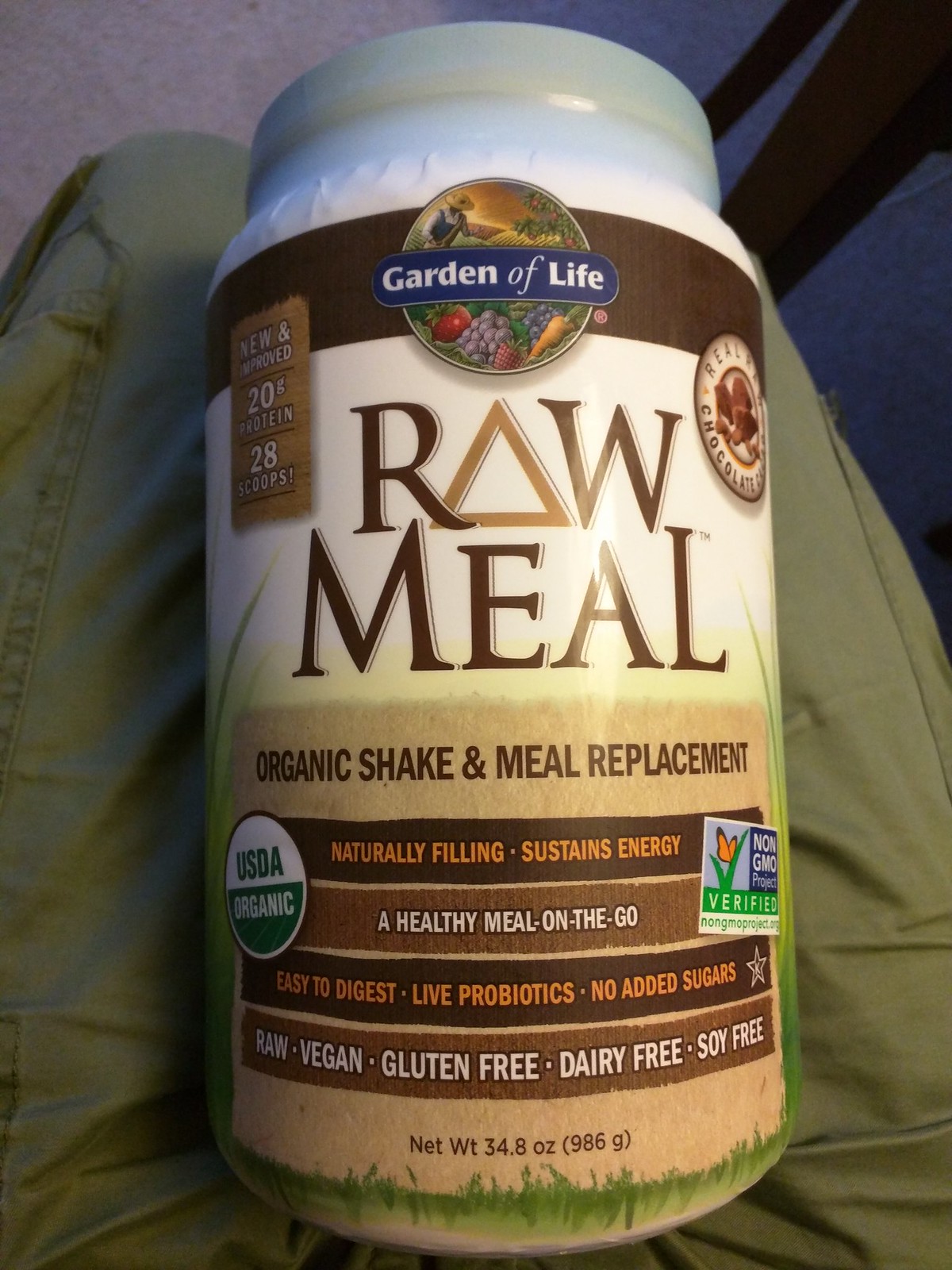This photograph captures a meal replacement bottle branded as "Garden of Life: Raw Meal." The white plastic container prominently features a brown and white label. The bottle is laying on someone's lap, with khaki pants visible in the background, suggesting a casual setting. At the top of the label is a circular emblem adorned with fruit, bearing the brand name "Garden of Life." Below this, the product name "Raw Meal" is clearly printed. On a brown background, the text reads: "Organic Shake and Meal Replacement." A circle, half white and half green, displays the "USDA Organic" certification.

Additional product details follow: "Naturally Filling, Sustains Energy, A Healthy Meal on the Go, Easy to Digest, Live Probiotics, No Added Sugars, Raw, Vegan, Gluten Free, Dairy Free, Soy Free." The net weight of the product is also indicated as 34.8 ounces (986 grams).